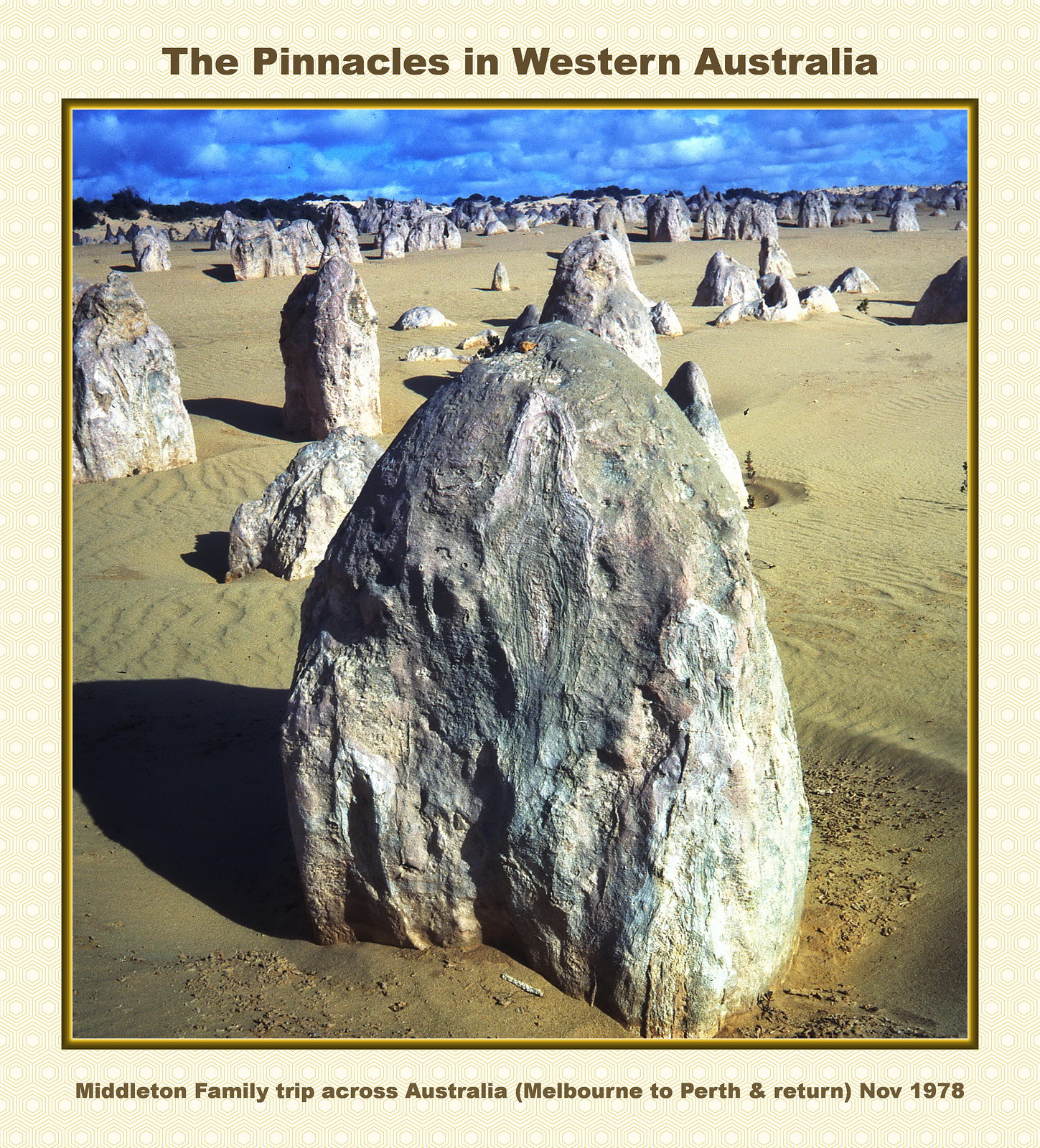The image appears to be a vintage photograph, possibly a postcard or a scrapbook entry, set against an off-white background with an outlined frame. The photograph captures the Pinnacles in Western Australia, showcasing a landscape filled with numerous sharp, pointed stone formations that extend to the horizon. These stones, about the height of a small person, cast long shadows across the sandy terrain. The sky is a vivid blue with clouds, giving the scene a slightly surreal, computer-generated appearance. The top of the image is labeled “The Pinnacles in Western Australia,” while the bottom text reads, "Middleton family trip across Australia (Melbourne to Perth and return), November 1978." The overall scene feels expansive, with hundreds, possibly thousands, of these unique geological structures spreading across the beach-like landscape.